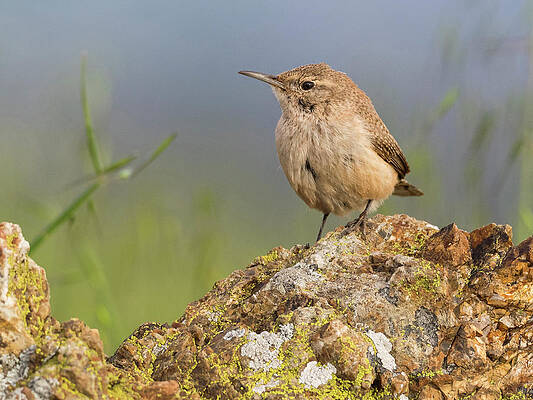This close-up photograph captures a small, light brown bird with touches of white feathering and subtle black markings. The bird has a slim, pointed beak and is standing on a jagged light brown rock, which features patches of green moss and some white areas. The bird, which appears regal in its simplicity, is positioned in profile, gazing to the right, with its left eye and beak sharply in view. The background is intentionally blurred, highlighting the bird and rock, but faintly reveals a mix of green vegetation and a dark blue sky, creating a serene and natural setting.